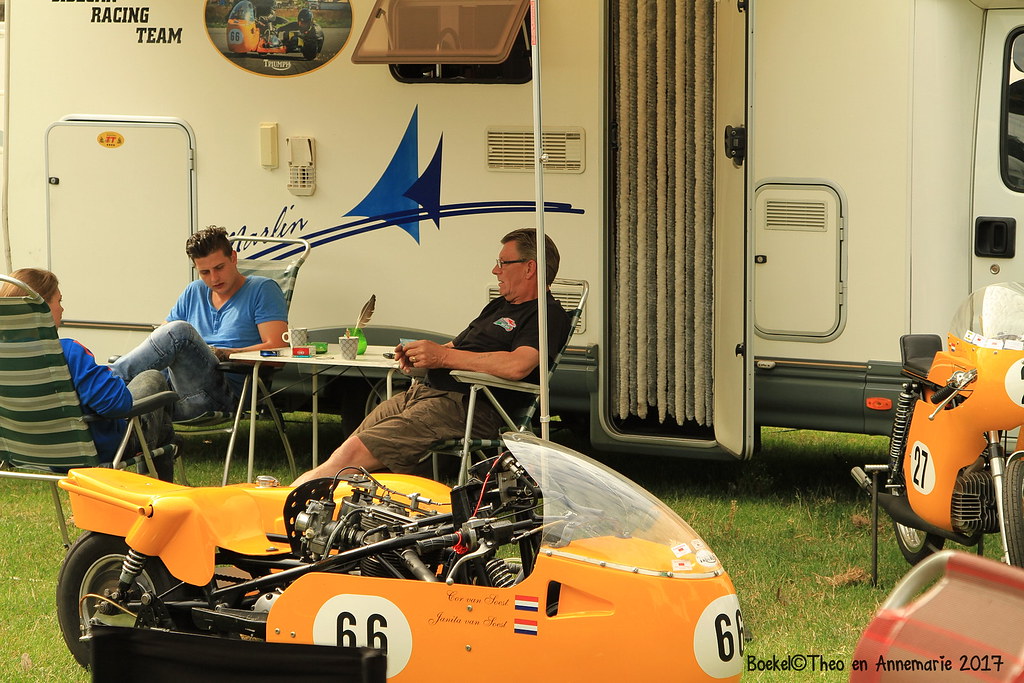This photograph captures a scene at a trailer park featuring a white camper with "Racing Team" written on it in black text. In front of the camper, there are three people sitting in lawn chairs. The man on the left is an elderly gentleman wearing glasses, a black shirt, and light brown shorts. To his right, another man sits in a light blue V-neck shirt and light gray jeans. On the far right, a third individual, possibly a woman, sits with their back turned to the camera. In the foreground, there are two striking orange racing motorcycles, both equipped with large screens. The motorcycle on the left bears the number 66, while the one on the right has the number 27 and includes a sidecar. Near the bottom right corner of the image, there is a watermark that reads "B-O-E-K-E-L" with a copyright symbol (©), followed by "Theo and Anne-Marie 2017."